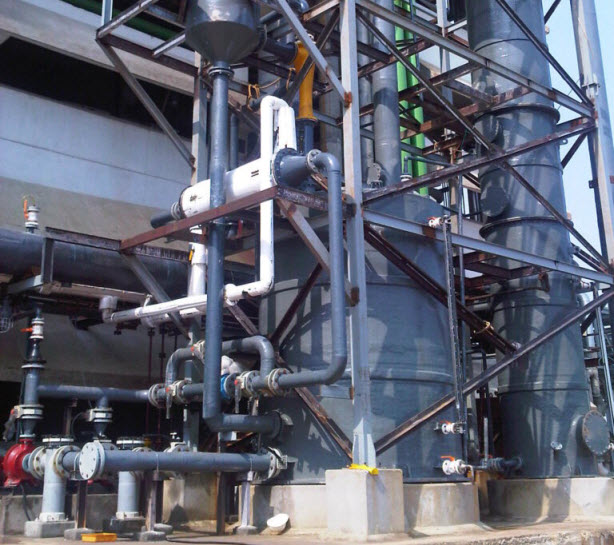This vertical photo captures a complex section of an oil refinery, showcasing an intricate network of blue and gray PVC piping. The pipes twist and turn at various angles, including 45-degree bends that form U-shapes, leading into a white and black pump. From the pump, the system continues through white tubing into a large cylindrical drum, perched atop a concrete foundation, capable of holding thousands of gallons. In the bottom left corner, a red pump connects to two pipes, adding to the intricate web of pipelines. The image is set outdoors with a clear sky visible in the background, hinting at the industrial scale of the refinery, surrounded by metallic structures and a distant wall.